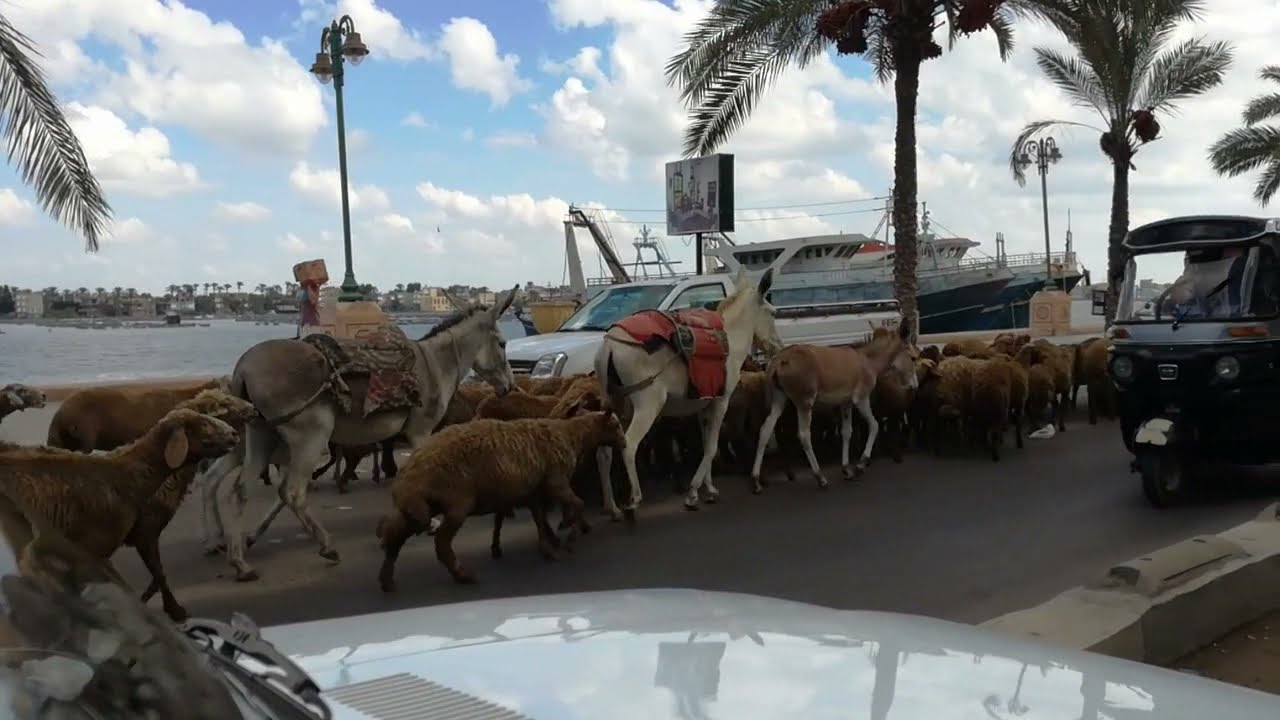The horizontal rectangular image depicts a lively scene set against a beautiful sky filled with fluffy white clouds and patches of blue. The top portion of the photo showcases this vibrant sky. Below, on the middle left, lies a body of water surrounded by buildings and land, with a large ship anchored in the harbor. 

Prominently in the center of the image, a bustling convoy of animals dominates a gray asphalt road. The convoy consists of three burros: a gray one, a white one in the middle, and a smaller light tan one in front, all connected by a rope. Accompanying them is a sizable herd of sheep, possibly around 15, marching along in a rather organized fashion. 

On the road, a black vehicle with a large driver window and a black top is visible on the middle right side, and the corner of the vehicle’s hood can be seen at the bottom of the image, reflecting light. Flanking the road, on the right side, is a light gray short stone wall, and further off in the background, power lines and a crane are noticeable.

Palm leaves hang slightly into the frame from the upper left corner, with more palm trees dotting the right side, adding a tropical feel to the setting. The colorful hues of blue, white, gray, green, brown, orange, and tan punctuate the scene, emphasizing the vibrant midday ambiance in what appears to be an Asian harbor town.